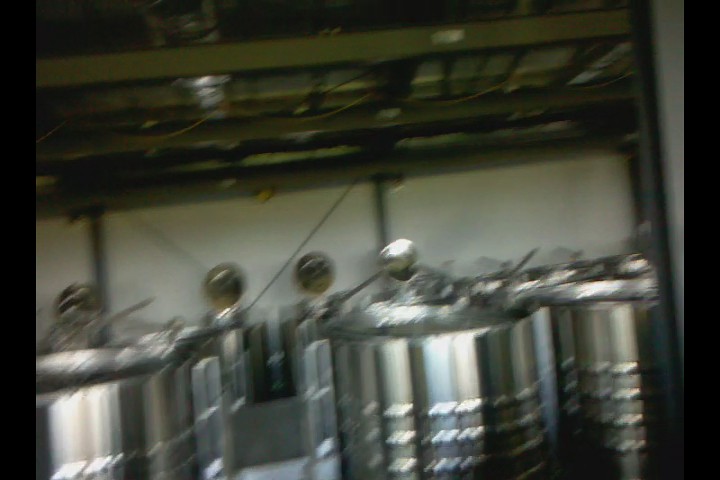The image is a very blurry photograph capturing a collection of shiny metal containers arranged on a dark grey, metal shelf. These containers, possibly stainless steel pots or pans, each feature distinctive cylindrical ribs or textures and reflect natural light that appears to come either from overhead or from behind the viewer. The containers seem to vary slightly in detail, with some potentially having open or crooked lids, suggesting an industrial kitchen setting. Despite the blur, a spoon or ladle is vaguely discernible atop one of the central containers. In the background, which includes a white wall, there are round, button-shaped objects and additional unidentified metal items. A straight black border runs vertically along both the right and left edges of the image from top to bottom.